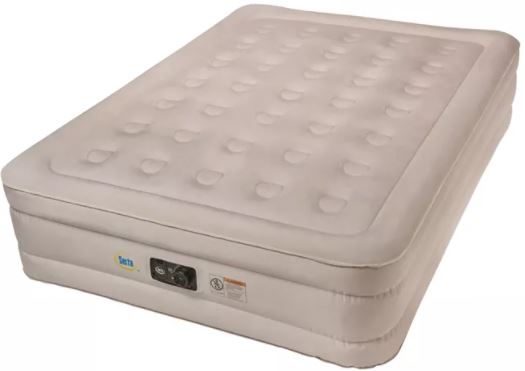This is a detailed photograph of a tan-colored inflatable mattress positioned on a clean white background. The mattress, a product of the Serta brand, features a padded, cushioned top dotted with 35 prominent circular indentations arranged in a grid of five columns by seven rows. The overall design of the mattress showcases a rectangular prism shape with rounded corners, and it is oriented slightly to the right, revealing both the top and the sides. The front side of the mattress displays several key elements: a small blue Serta logo on the left, a larger black label with white text and image in the center, and an instruction sticker incorporating black, white, and orange elements to the right. Additionally, there is a black connection port centrally located, intended for attaching a pump to inflate the mattress. The sides are detailed with two horizontal seam lines that circumnavigate the mattress, adding both structural support and aesthetic definition.